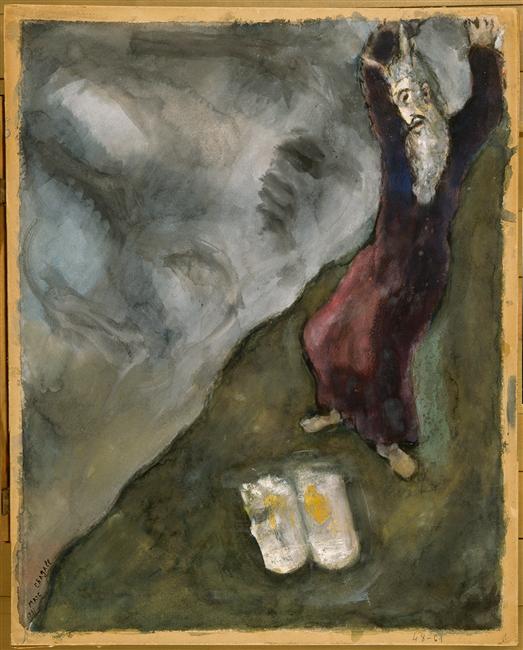The painting, which appears to be "Moses Breaks Tablets of Law 1931," is a detailed and abstract portrayal of a reclining elder man. The man, likely representing Moses, is situated on the right side of the image, against a dark green surface accented with black. He has a flowing long gray beard and is barefoot, with his feet in front of him on a brownish area. Moses is dressed in a dark burgundy or maroon tunic-like robe. His eyes appear to be closed, suggesting a state of contemplation or possibly death, and his arms are raised above his head.

At his feet are two white, rounded objects with golden splotches, likely representing the tablets of the law. The left side of the painting features a swirling, stormy sky composed of white, gray, and black hues, creating a foreboding atmosphere. The image is bordered by a thin yellowy-gold outline, which frames the entire scene. The artist's name and an unreadable date are inscribed in the bottom right corner, adding a signature touch to this profound and thought-provoking artwork.